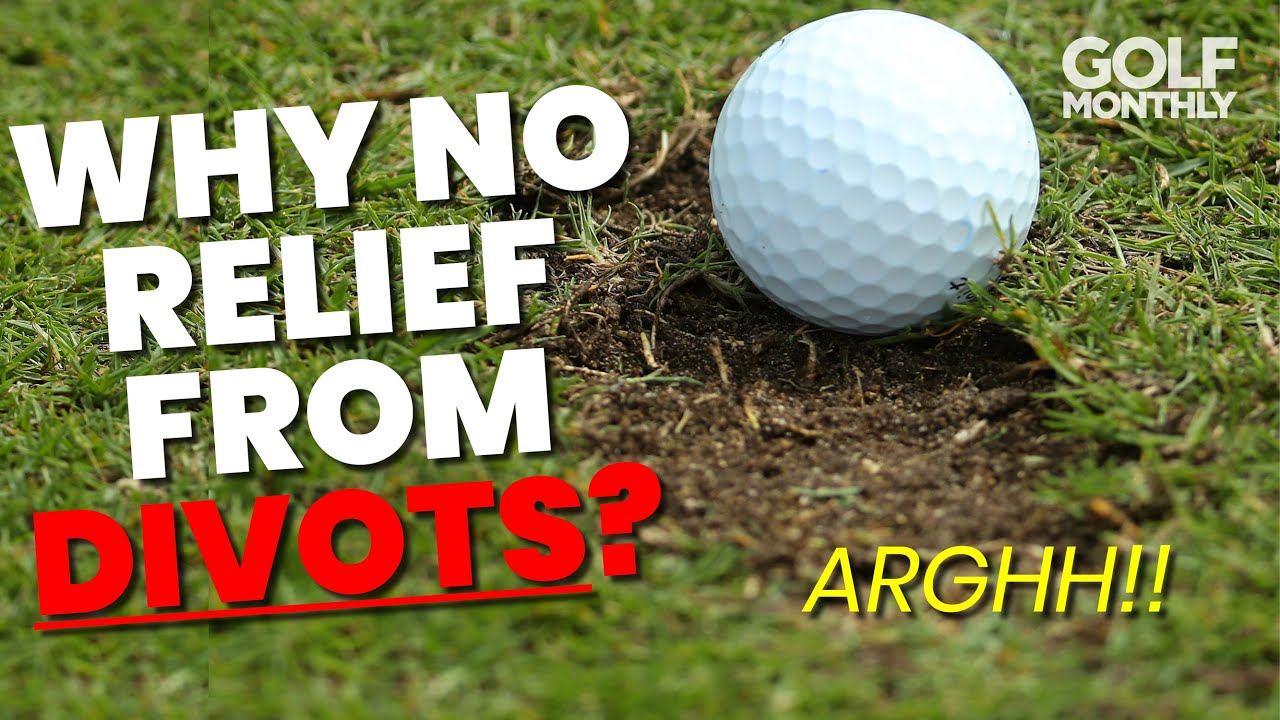The image, likely a cover of Golf Monthly magazine, features a white golf ball set on a well-manicured, green golf course. The ball lies in a divot made from a golf club, surrounded by short grass with the exposed brown dirt of the divot directly in front of it. The scene is in sharp focus in the middle, while both the foreground and background are slightly blurry. In the upper right corner, there is semi-transparent white lettering that reads "Golf Monthly." To the left, bold text exclaims "Why No Relief from Divots?" with "Divots?" underlined in red, and a frustrated "ARGH!!" highlighted in yellow to its right. The overall composition emphasizes the clear, untouched state of the golf ball amid the challenging condition of the divot, engaging the reader in the common frustrations experienced on the golf course.